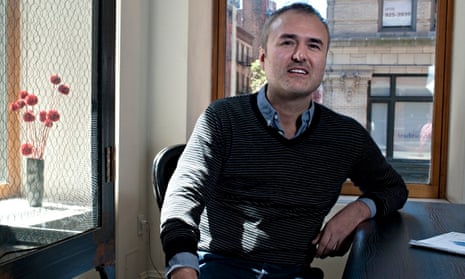The detailed photograph depicts a man of European descent seated in a corner of a sunlit office with white walls and a tan corner wall. He is situated in a black office chair at a dark charcoal-colored desk or table, facing the camera directly. The man's left arm is bent at the elbow, resting on the table with his hand dangling off the edge, while his right arm extends outward with his hand placed on his right knee. He appears to be in his late 30s to mid-40s, with a mix of graying brown hair, an oval face, and slight stubble. He wears a blue, slightly unbuttoned button-down shirt under a dark-colored sweater with horizontal black and gray stripes. 

To his left (the photo's right), there's a cabinet with a chicken wire-style door, containing a vase filled with long-stemmed red pom-pom shaped flowers. Adjacent to the cabinet is an artwork in a black frame, showcasing a tall, slim white vase with pink flowers on a white table against a white background. Behind the man is another artwork or possibly a window with a light brown wooden frame that offers a view of a cityscape featuring old limestone buildings and a modern high-rise with black trim. Through this window, one can see various buildings including old stone structures with decorative garlands and modern red brick buildings. The office appears orderly with the man seemingly focused or just having turned to acknowledge the photographer, giving a slight smile as if engaged in conversation.